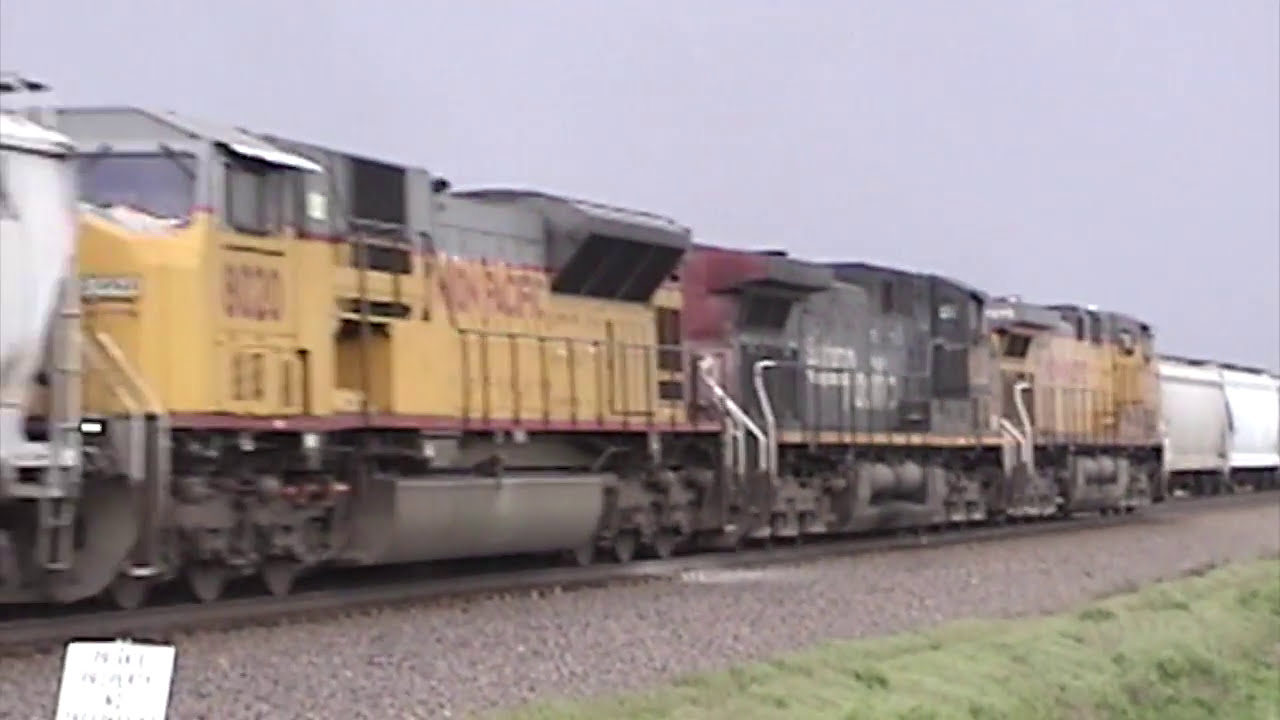This image is a color photograph showcasing a line of three modern locomotives traveling through an outdoor area. The leading locomotive is yellow with a gray top and bottom, and the one behind it is gray with red accents. Another yellow locomotive is linked behind these. Each locomotive has visible side railings and mechanisms, and they are traversing steel tracks laid over a bed of gravel. Attached to these locomotives are several train cars, including white tank-like cars. For added context, there is greenery and gravel in the lower right corner of the frame, and the background features a mostly gray sky. The image quality suggests it is a screen grab from an older, lower-resolution video.